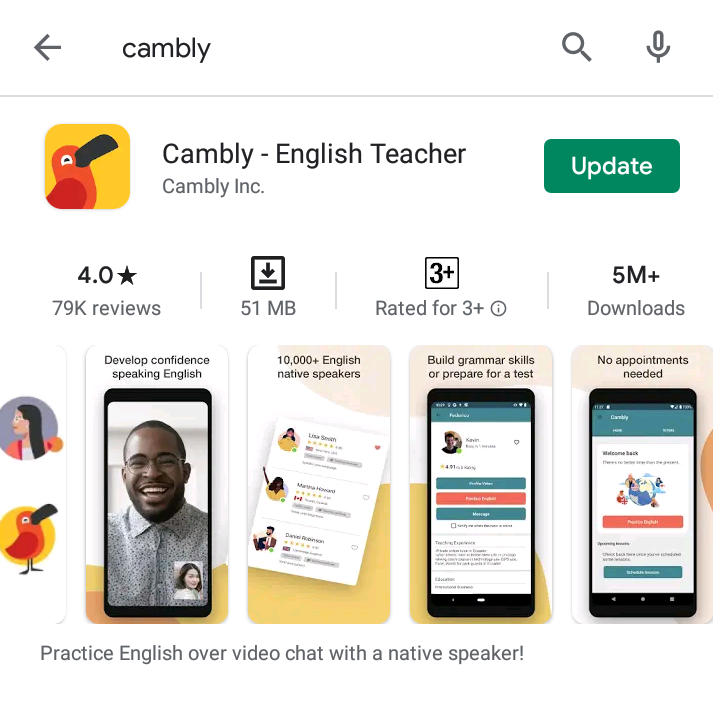This is a detailed caption provided for a screenshot of the "Cambly" app from the Google Play Store app page:

The screenshot features the "Cambly" app information page within the Google Play Store interface. The background is predominantly white. At the top, there is a navigation bar with an arrow pointing to the left on the far left, followed by the app name "Cambly" in lowercase black letters. To the far right, the navigation bar includes a search icon (magnifying glass) and a microphone icon. Below this bar, a light gray horizontal line, approximately 1-2 pixels thick, separates the top section from the rest of the app details.

The app icon, located below the navigation bar, is a square with rounded corners and a yellow background featuring a red illustrated toucan in a side view, sporting a black beak and gazing upwards. To the right of the app icon, text reads "Cambly – English Teacher" followed by "Cambly Inc." Beneath this text is a green button with rounded corners and the word "Update" in white letters, indicating that the app is installed and an update is available.

Following the app icon and name section, there are additional details organized into columns:
- The first column shows a 4.0-star rating.
- The second column indicates "79K reviews".
- The third column displays a download size of "51 MB" with an icon of a box and an arrow pointing down.
- The fourth column shows "3+" within a square, indicating the app is rated for ages 3 and up, accompanied by an information icon.
- The fifth column notes "5M+" downloads.

Below these columns, there are five preview images of the app:
1. The first image, partially cut off, depicts an illustrated woman alongside the app's bird logo.
2. The second image showcases the app's interface with the text "Develop confidence speaking English" and features a phone template with a man talking to a woman in the bottom right corner.
3. The third image highlights "10,000+ English native speakers" with a visual of reviews.
4. The fourth and fifth images provide further previews of the app functionalities.

Below the images, text reads "Practice English over video chat with a native speaker," summarizing the app's purpose.